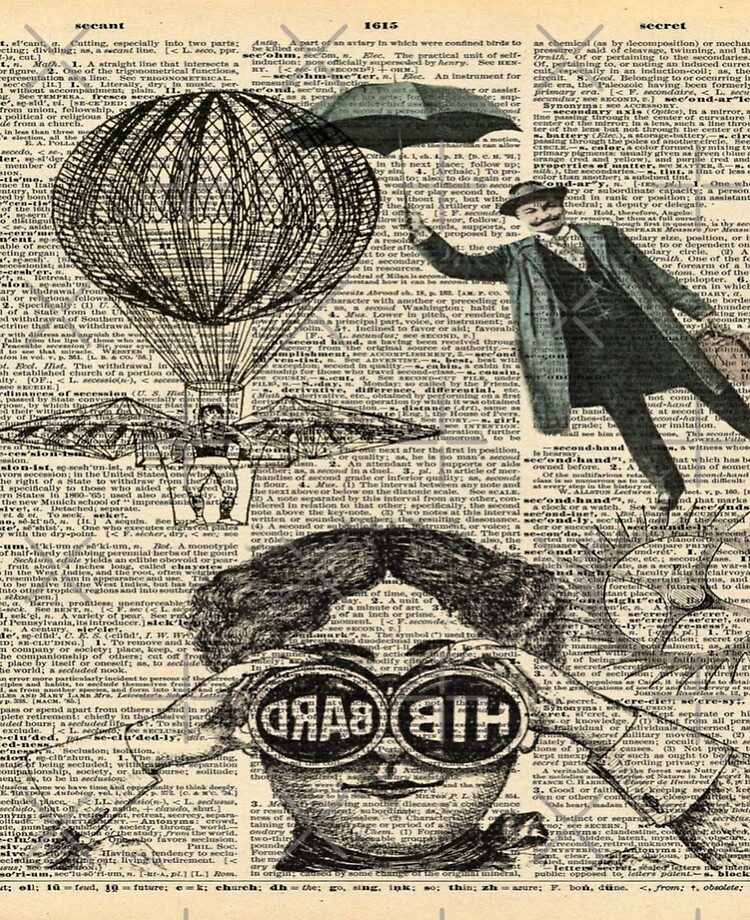This picture appears to be an aged, tan newspaper or dictionary clipping divided into three columns of small, dense, and mostly illegible text. In the upper left corner, the heading "Secants" appears, similar to a dictionary entry with definitions and descriptions related to the term "math." Centralized at the top is the number "1615," and the top right is titled "Secret." Overlaying these columns are intricate black and white illustrations: 

On the left, spanning over the left and middle columns, a detailed drawing features a hot air balloon with a man navigating it, equipped with wings extending from the sides of the platform. 

Towards the top right, a man dressed in a black suit, holding an umbrella, and sporting a top hat, is depicted as if standing over the text. 

At the bottom of the page, an illustrated face with short, curly hair parted in the middle is shown gazing through a pair of binoculars, with the name "Hibbard" appearing backward beneath this image.

The entire tableau gives a surreal and vintage feel, accentuating the sense of historical intrigue matched with imaginative art.